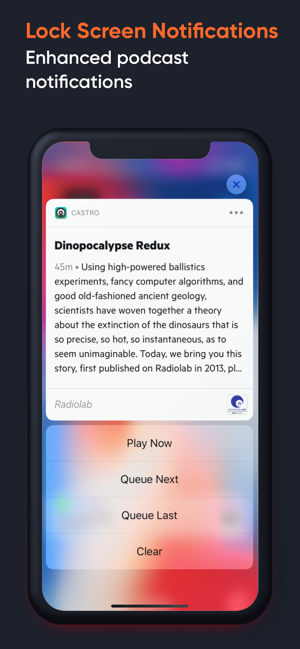The image depicts an advertisement for a mobile application focused on enhanced podcast notifications. The header, rendered in bold red text with capitalization on significant words, reads "Lock Screen Notifications." Directly beneath it, in a smaller font, is the subheading "Enhanced Podcast Notifications."

Centrally featured is a smartphone displaying a notification interface. Prominently, the notification header bears the name "CASTRO" in all capital letters next to a symbol consisting of a circle with a dot inside it. To the right of this header are three horizontal dots, indicating additional menu options.

Below the header, the notification details are displayed. The title "Dino Apocalypse Redo" stands out, presented in capitalized "D" and "R." Accompanying the title is the duration "45 minutes" in a subdued light gray font. The detailed description follows, stating: "Using high-powered ballistics, experiments, fancy computer algorithms, and good old-fashioned ancient geology, scientists have woven together a theory about the extinction of dinosaurs that's so precise, so hot, so instantaneous as to seem unimaginable. Today we bring you this story, first published on Radio Lab in 2013." The mention of "Radio Lab" is accompanied by its logo.

At the bottom of the notification are four interactive options: "Play Now," "Cue Next," "Cue Last," and "Clear," allowing users to manage their podcast listening experience directly from the lock screen.